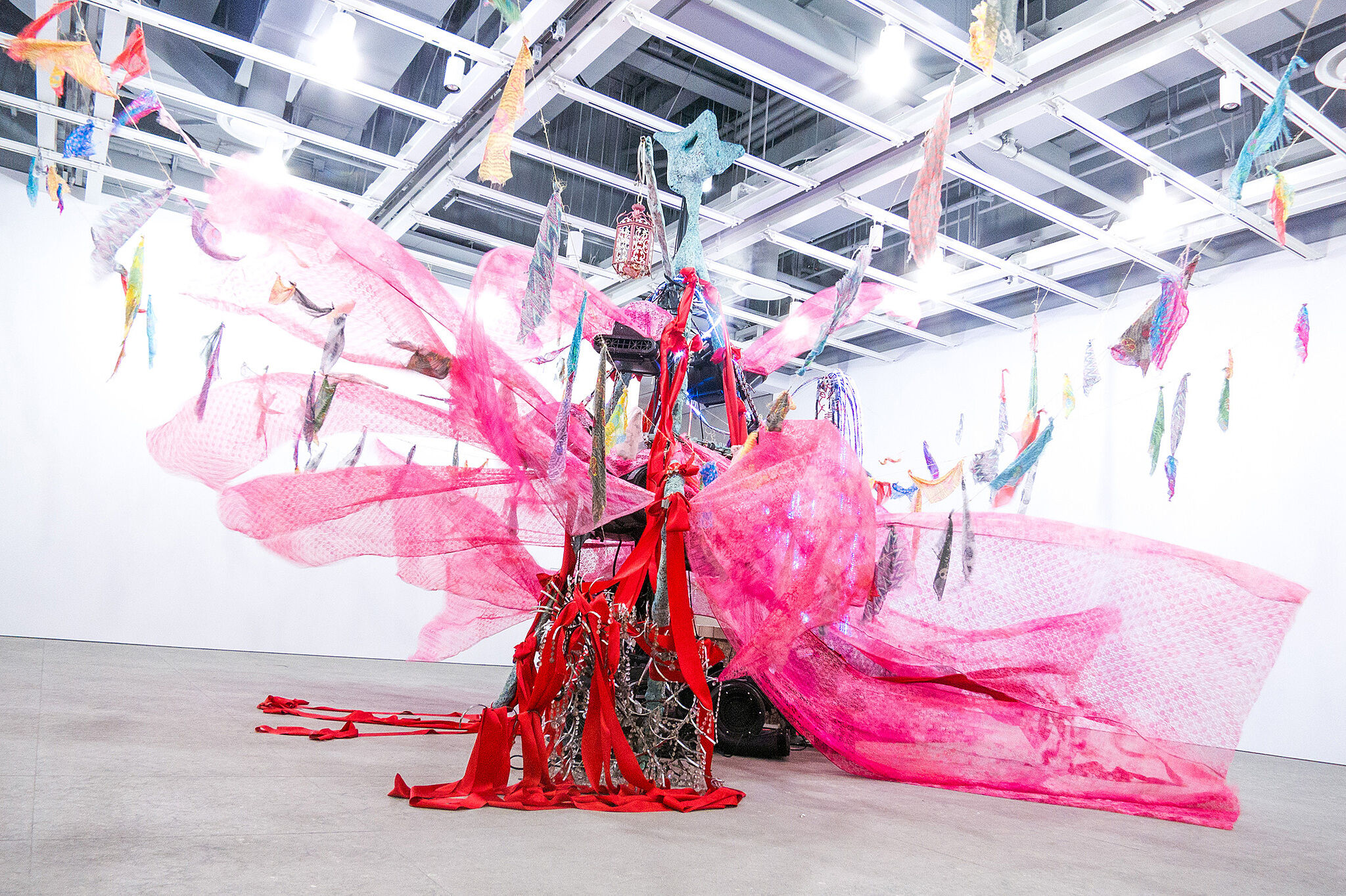The image depicts an art museum exhibit situated in an industrial room with a concrete, gray floor and white walls. The ceiling is open and unfinished, revealing metal grates, HVAC units, lighting, and various piping systems. The focal point is a large, intricate installation hanging from the ceiling, consisting of pink sheer material prominently draped and tied into a bow. Interwoven with this pink netting are vibrant, multi-colored pieces of fabric, including shades of orange, yellow, blue, and red. These fabrics are fastened in an arc-like pattern from one portion of the ceiling to another, accompanied by thick red string and silver chains. Additionally, the exhibit includes various silver metal artworks, red ribbons, a chandelier, and a blue star positioned at the top. The overall impression is a complex and colorful display blending textiles and industrial elements in a captivating manner.